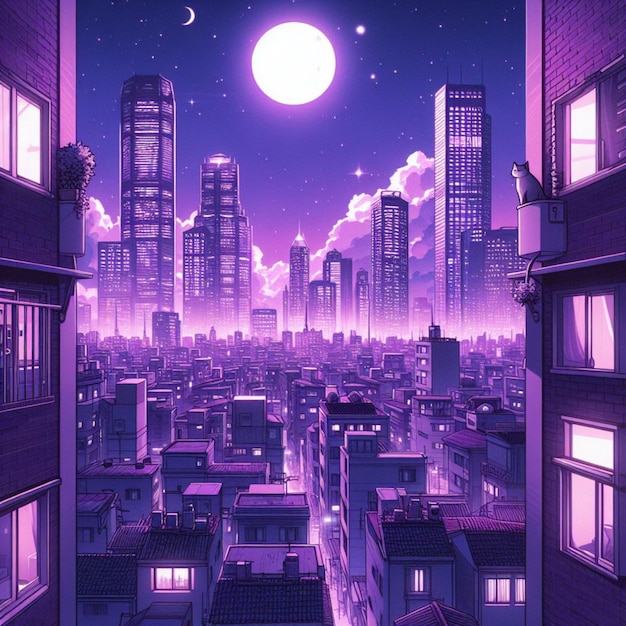This digital rendering depicts a bustling urban cityscape at night, dominated by tones of purple and blue. Flanking the image on the left and right are brick buildings each with three windows across three stories. The right building features an upper-story window with a white cat perched on what appears to be an electrical or utility box, while the left building showcases a flower box beneath its top window. Below, an overhead view reveals a sea of shorter, rectangular buildings with illuminated windows extending into the distance. Towering in the background are extremely tall skyscrapers, their countless windows glowing against the night sky. Above these structures, billowing clouds mingle with a sky speckled with white stars. A large glowing white orb, possibly a moon, dominates the center, accompanied by a smaller crescent moon on the left and another smaller glowing orb on the right, adding a layer of surrealism to this nocturnal cityscape.